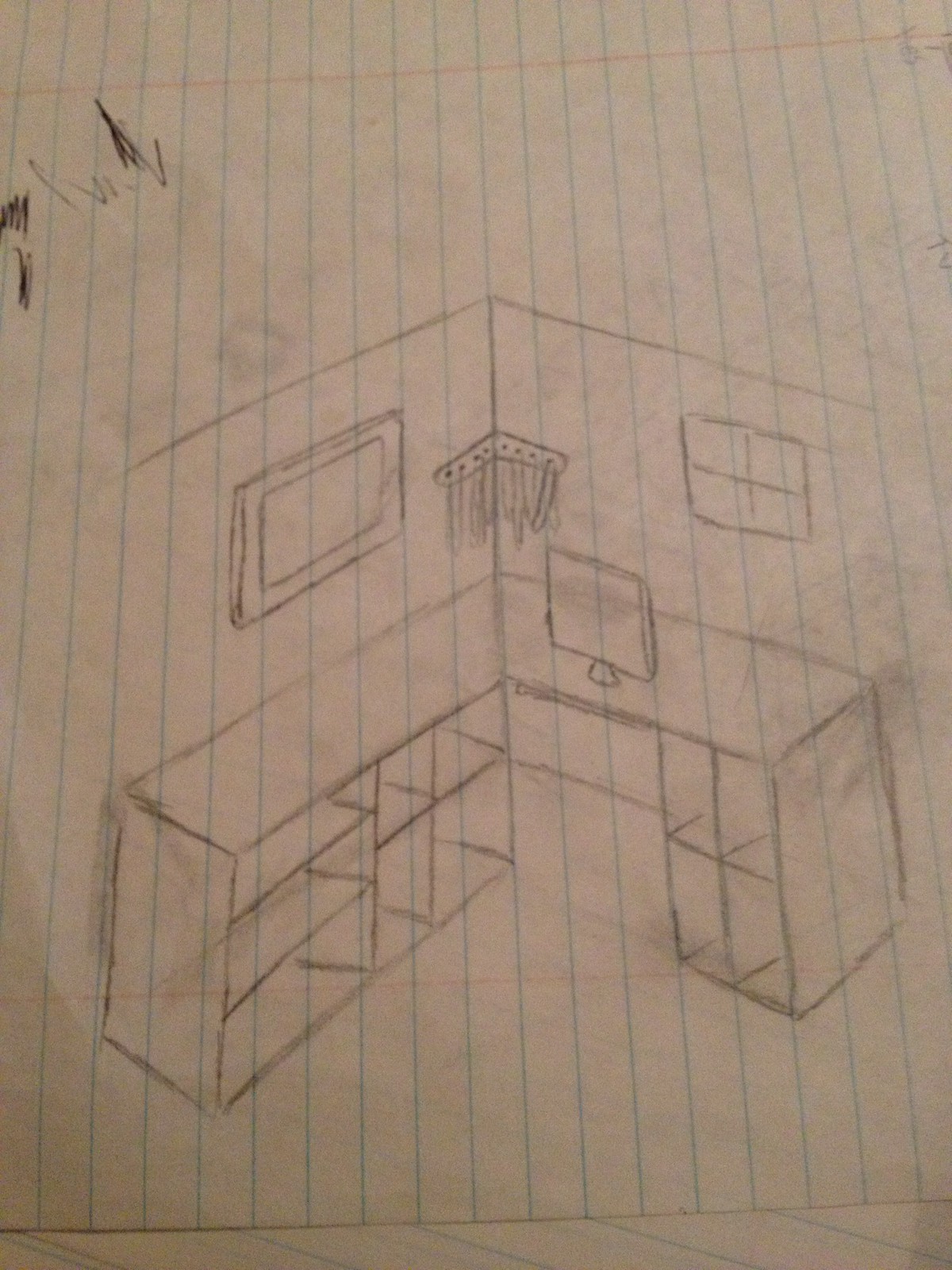This image is a detailed pencil drawing on lined notebook paper, showcasing a 3D perspective design for a home office. The drawing spans two walls that form a corner, supporting an L-shaped desk. One side of the desk features shelving suitable for books and other storage, while the other side has cubby holes and cabinets. A computer monitor sits on the desk, drawn simply without additional peripherals. One wall includes a framed picture, and the other wall features a window. Blue horizontal lines cover the notebook paper, with distinct red lines at the top and bottom margins, and some scribbles in the top left corner. The detailed rendering, with thoughtful consideration of desk functionality and wall adornments, suggests it might be a school project by a child.